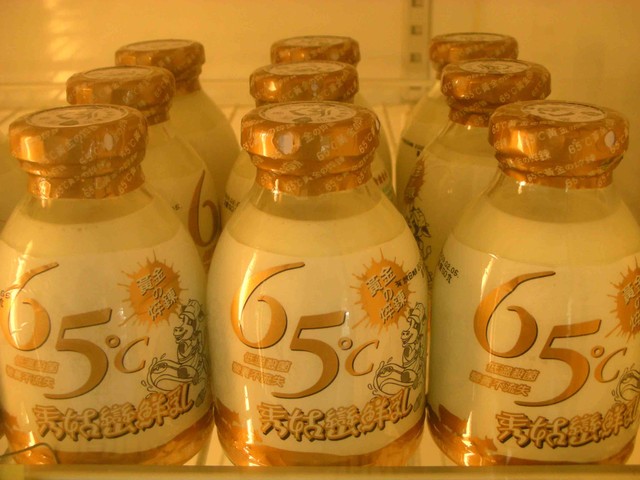This image, taken inside a refrigerator, shows a close-up of nine small, round glass bottles arranged in three rows of three on what appears to be a glass shelf, as indicated by the subtle reflection at the bottom of one bottle. Each bottle contains a white, milky liquid and features a gold color on both the lid and the wrapper. The front of each bottle is marked with "65 degrees Celsius" and displays a picture of a cow, along with some Chinese or Japanese writing. The entire scene has a yellowish or orange tint, possibly due to the refrigerator's interior lighting. Behind the bottles, the white wall of the fridge and some metal structures, including a horizontal line and a vertical piece with squares, are visible.